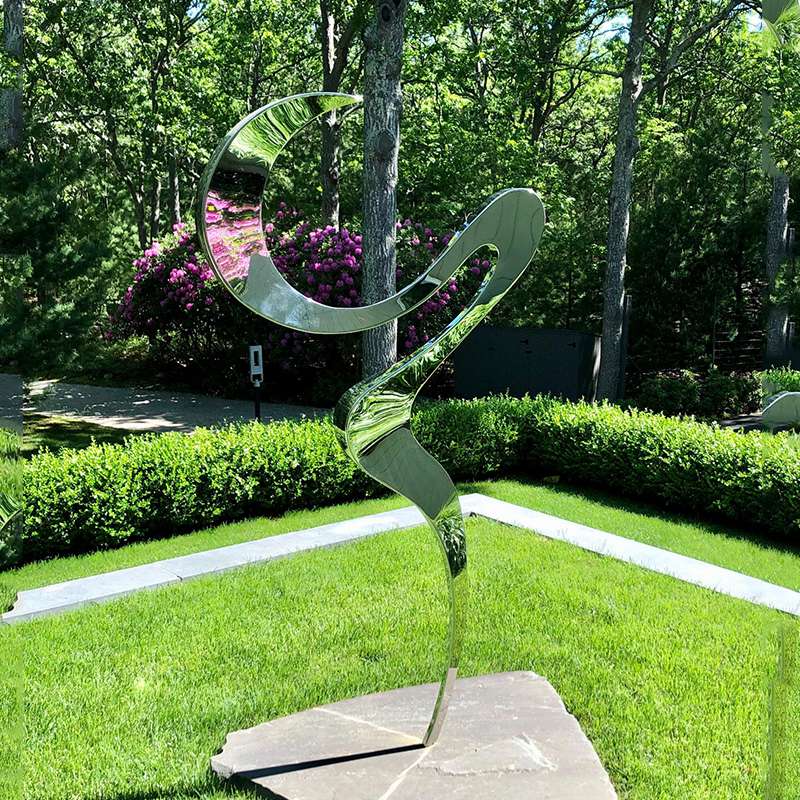In the center of this grassy area framed by concrete, there stands a striking piece of public art. It's mounted on a stone slab and features a highly reflective, mirror-like surface. The artwork itself forms an elegant, twisting line that starts thin and gradually widens, culminating in a series of curves that almost form a letter C. This sinuous shape catches and reflects the surroundings, adding to its captivating presence. Encircling the grassy square is a low hedge, and just beyond this lies a pathway. The background is lush with large trees and dense foliage, interspersed with vibrant purple flowers, creating a serene and picturesque environment that enhances the beauty of the display. This peaceful, natural setting makes it an inviting place for a leisurely walk while appreciating the interplay between art and nature.